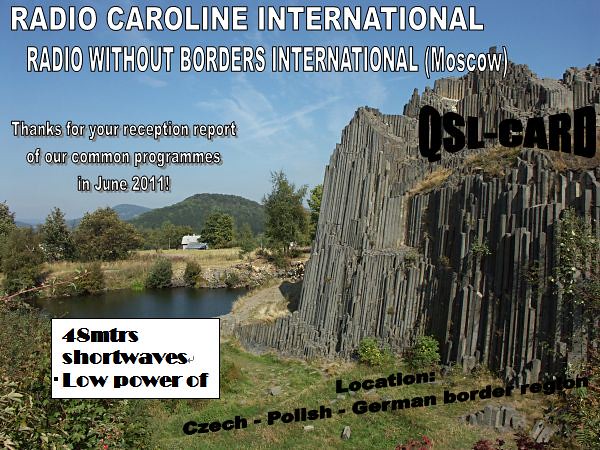The photograph showcases a unique and fascinating landscape featuring oddly-shaped cliffs that resemble vertical sticks or stalactites, with the brown, thin, blocky formations creating a jagged appearance as they protrude towards peaks. In the background, there's a small body of water on the left, with grassy fields and several houses visible, leading to a distant, green-covered mountain range. The sky above is blue adorned with wisps of clouds. Superimposed on the image is white text that reads: "Radio Caroline International, Radio Without Borders International (Moscow). Thanks for your reception report of our common programs in June 2011." Additionally, a white text box located at the bottom left of the photo contains the inscription, "48 MTRS, short waves, low power of," while the bottom right corner provides the location details: "Czech-Polish-German border region." This QSL card celebrates international radio communications and acknowledges listener feedback.